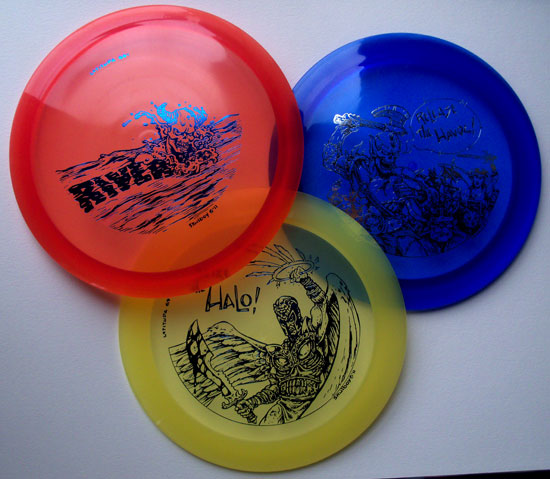This photograph, taken from a top-down perspective, captures three semi-transparent frisbees overlapping slightly on a plain white surface, which gives a subtle greyish hue. The frisbee on the upper left is red and features a water wave design in blue along with the word "river." The top right frisbee is blue and showcases a scene with warriors in armor, one of them holding an axe, though the text is illegible. The bottom middle frisbee is yellow, adorned with the word "HALO!" and a detailed illustration of a masked, armored figure with wings, wielding a sword and holding a crown with feathers in one hand.